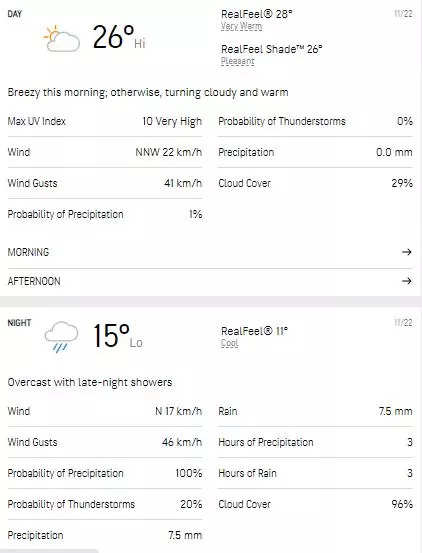This image depicts a detailed weather chart divided into two sections: daytime at the top and nighttime at the bottom. 

**Daytime Weather:**
- In the top-left corner, a sun partially obscured by a cloud indicates the weather for the day with a high temperature of 26 degrees Celsius.
- To the right, "Real Feel" temperature is stated as 28 degrees Celsius, with a shaded "Real Feel" also at 26 degrees Celsius.
- Below these details, it mentions: "Breezy this morning, otherwise turning cloudy and warm."
- The left side lists key weather statistics including:
  - Maximum UV Index
  - Wind speed
  - Wind gusts
  - Probability of precipitation
  - Probability of thunderstorms
  - Precipitation
  - Cloud cover

**Nighttime Weather:**
- The bottom section displays a cloud with rain, indicating the nighttime weather, with a temperature of 15 degrees Celsius.
- To the right, "Real Feel" is noted to be 11 degrees Celsius.
- On the left, it states: "Overcast with late night showers."
- Nighttime weather details are listed in two columns:
  - Wind speed
  - Wind gusts
  - Probability of precipitation
  - Probability of thunderstorms
  - Precipitation
- Additional details include:
  - Hours of rain: 3 hours
  - Cloud cover: 96%

The chart offers a comprehensive outlook on both the day's and night's weather conditions, making it useful for detailed planning.